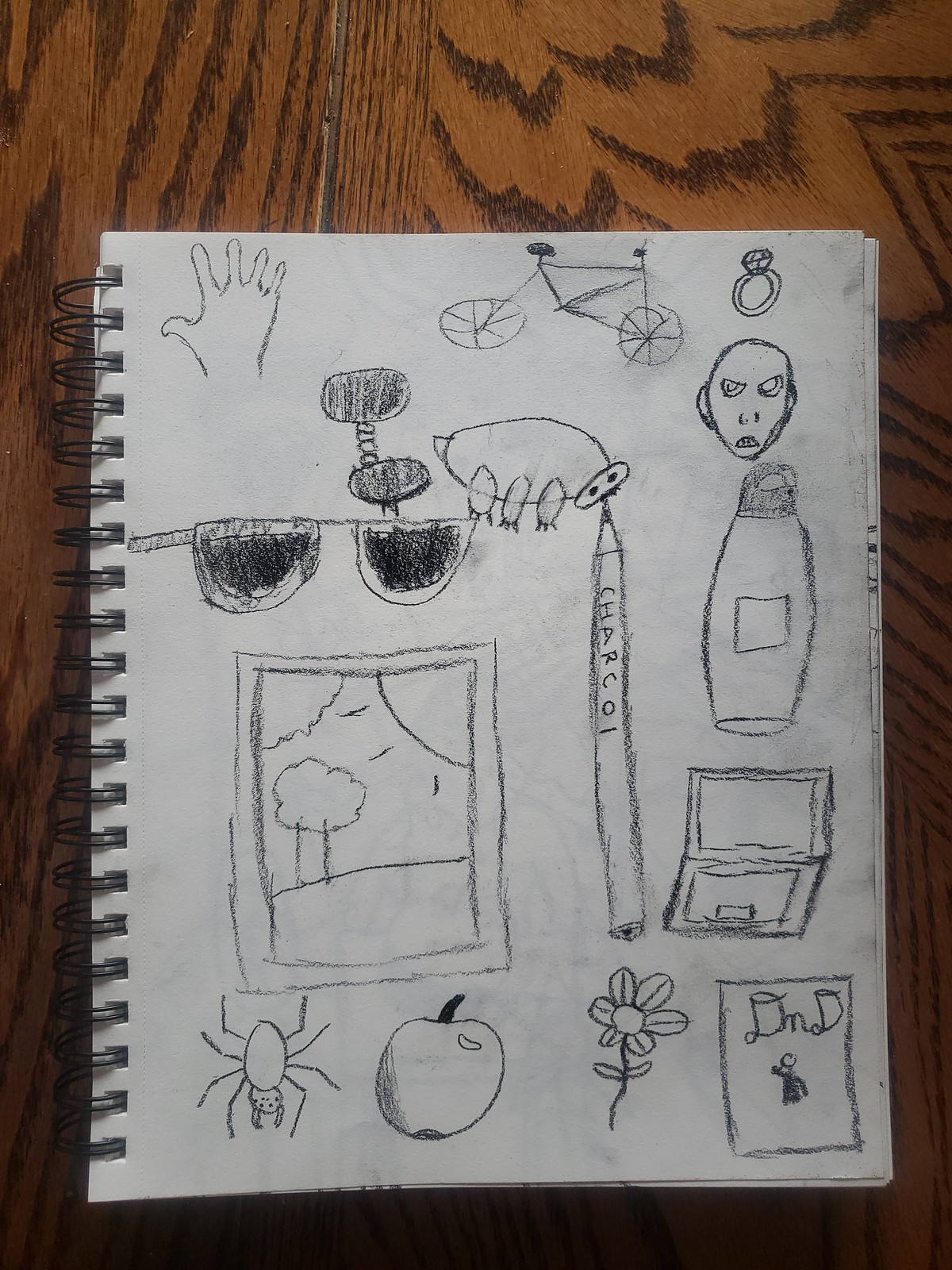The photograph depicts a page from a spiral-bound sketchbook resting on a brown wooden surface with a charcoal-like grain, possibly faux wood or veneer. The paper is upright and rectangular, and all the illustrations appear to be drawn in pencil.

Starting from the top, there is an image of a right-hand blade left open. To its right is a simple bicycle sketch, followed by a drawing of a diamond ring. Directly below these, there's an indistinguishable sketch. Adjacent to it is a depiction of an animal with three front legs and an oval head. Next to it is a face with a sneering expression.

Below the face, on the left, are dark sunglasses. Continuing downwards, there is a sharp-pointed pencil labeled "charcol" (intentionally misspelled as C-H-A-R-C-O-L). To the right of this pencil is a bottle with a square label and further to its right is an open laptop.

Returning to the left side, underneath the sunglasses, there is a drawing of a window showcasing the sun, clouds, and a tree. Below this window is a spider. Adjacent to the spider, on the right, is an apple, followed by a flower. Lastly, to the far right is a square with the cursive letters "dNd" and a figure of a person underneath.

Each sketch is carefully drawn, juxtaposing various objects and scenes, creating a whimsical and detailed collage on a single page.